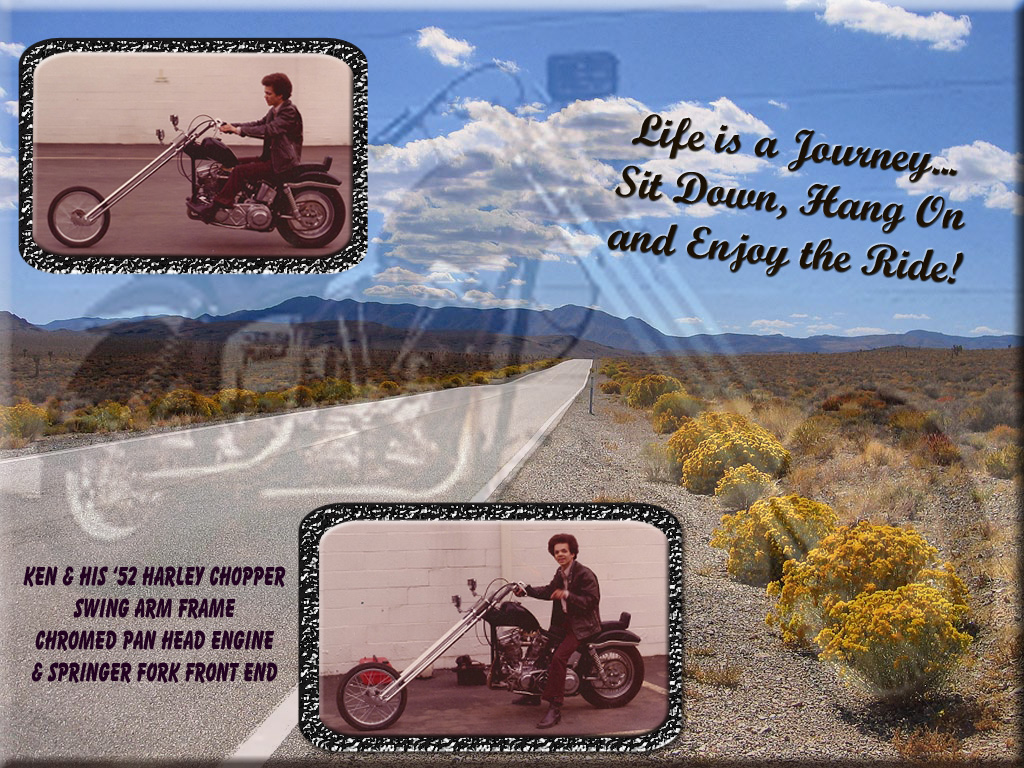The image resembles a postcard featuring an open, empty highway stretching into the distance with mountains in the background, set against a vibrant blue sky filled with puffy clouds. Superimposed on this scenic backdrop are two smaller photos of a man riding a distinctive 1952 Harley chopper; in the upper left, he is seen driving the motorcycle to the left, and in the center-bottom, he is sitting still on the motorcycle with his feet on the ground. The chopper is noteworthy for its extended front wheel, angled at 45 degrees, similar to an "Easy Rider" style. In the sky area on the right, a motivational quote reads, "Life is a journey. Sit down, hang on, enjoy the ride." In the lower left of the image, text details the motorcycle’s specs: "Ken and his '52 Harley chopper, swing arm frame, chromed pan head engine, and Springer fork front end." The overall composition suggests it could be an advertisement for the motorcycle, with colors including blue, white, gray, tan, black, yellow, green, and red contributing to the lively, outdoor, midday setting.